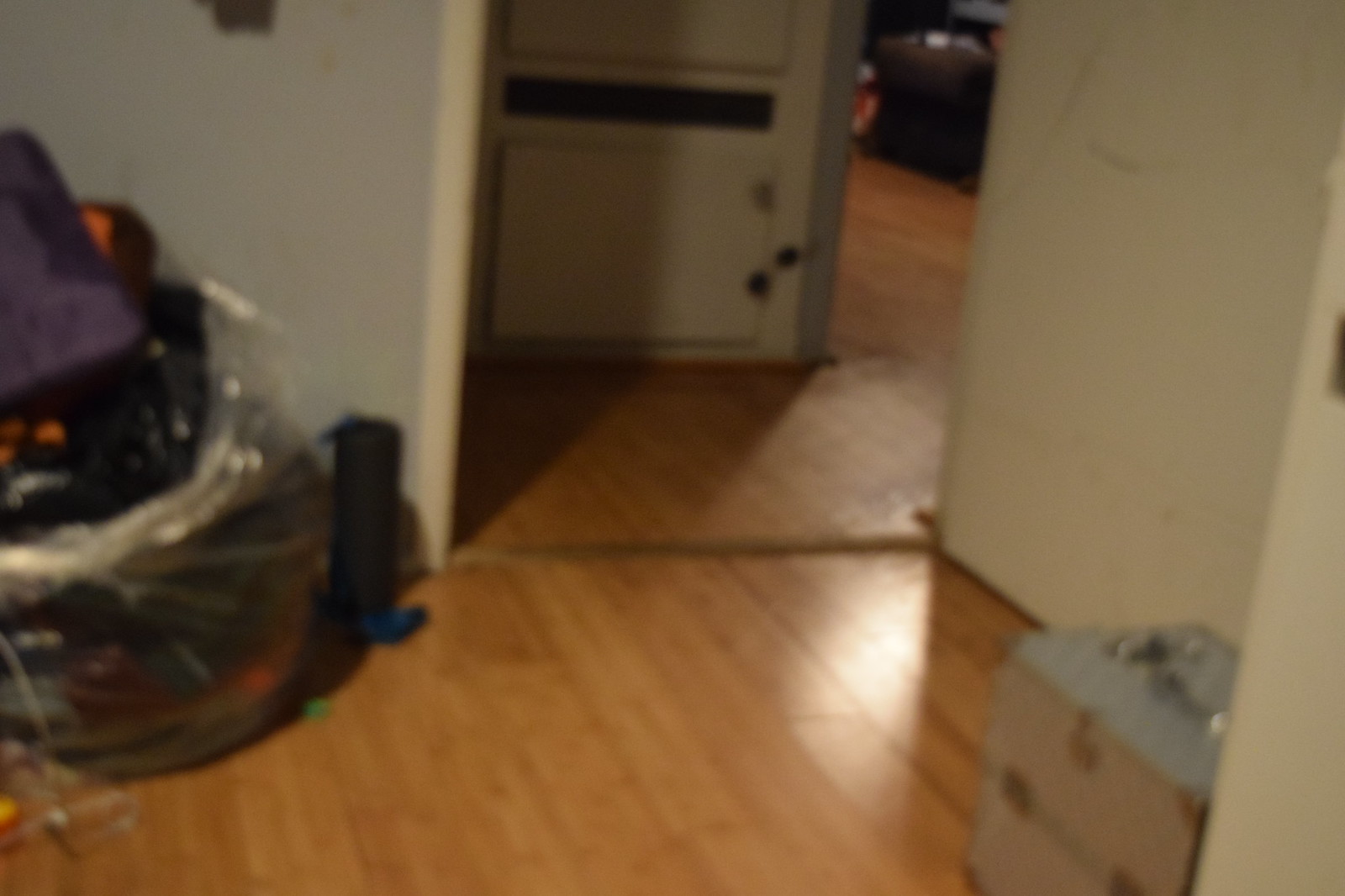The photograph captures a hallway within a home’s living area. The walls are predominantly white, with a section of a wall starting in the bottom left-hand corner. Resting on the light brown wooden floor is a small gray suitcase. To the right, another wall, in an off-white hue, displays some minor markings. Scattered on the floor are clear plastic bags containing various items in blue, purple, and orange, though the specifics are indistinct. The scene transitions into another room through a doorway framed with white trim. Beyond the doorway, the wooden flooring continues into the next room, where you can glimpse some brown furniture against the white walls.